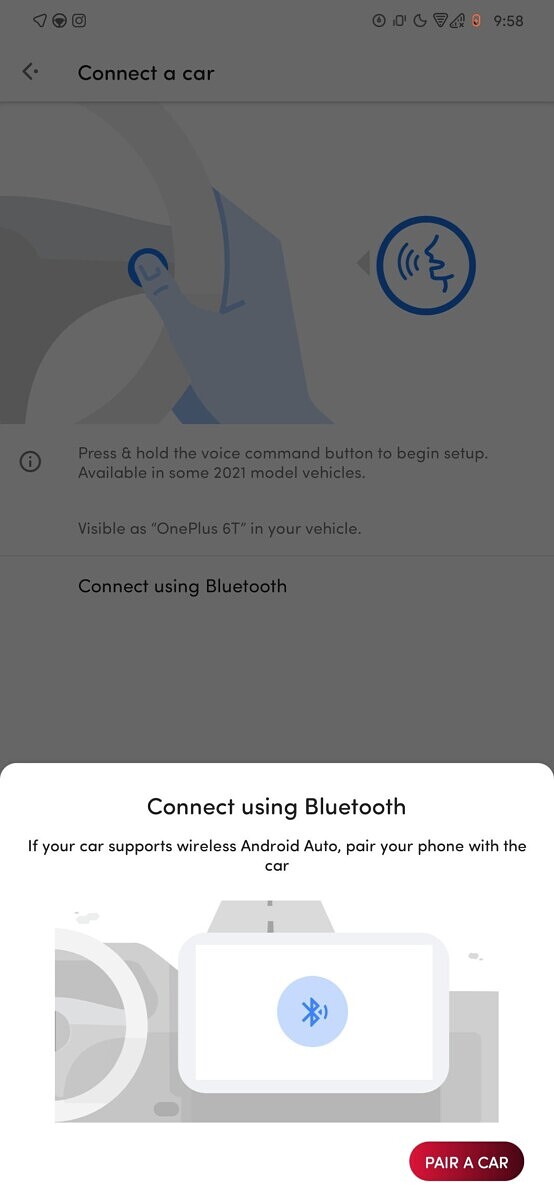The image displays a long, vertical, rectangular interface on a user's smartphone screen. At the very top, the time is displayed as 9:58. Directly beneath the time, there is a header with a back arrow and the text "Connect a car" in black. Below this header, a graphic illustrates a light blue hand gripping a gray steering wheel. Adjacent to the graphic, on the right, is a bright blue circle containing a white silhouette of a person speaking. 

Further down, brown text provides instructions: "Press and hold the voice command button to begin setup, available in some 2021 model vehicles." Following this, additional information in black text reads: "Visible as OnePlus 6T in your vehicle." Right below, another prompt states: "Connect using Bluetooth."

Overlaying this entire screen is a somewhat translucent dialogue box appearing at the bottom. This white box contains a message: "Connect using Bluetooth. If your car supports wireless Android Auto, pair your phone with the car." To support this instruction, there is an image of a cell phone next to a steering wheel, followed by a prominent red button labeled "Pair a car" in white text.